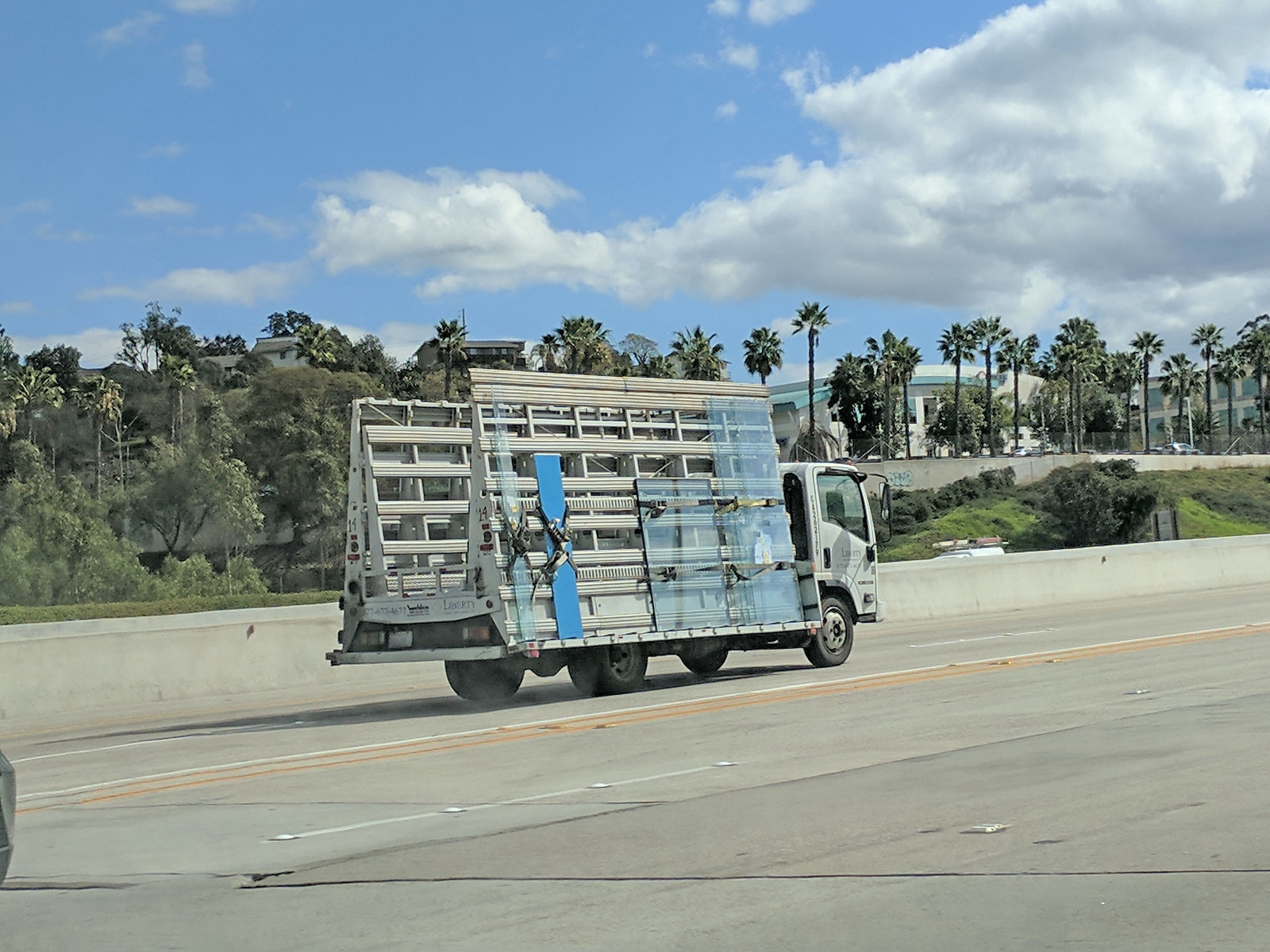This detailed color photograph taken outdoors in daylight features a white truck with a tall, metal-framed bed carrying large panes of glass, secured with a blue strap or board. The truck, which has a square cab design, is driving on a wide, multi-lane highway from left to right. The highway is gray with yellow and white dividing lines, and a concrete barrier separates the lanes. The sky is a bright, light blue adorned with fluffy white clouds concentrated towards the right side. In the background, there are numerous tall palm trees and a distant building partially obscured by foliage. Additionally, some elevated houses surrounded by greenery can be seen peeking through the trees, suggesting a warm location reminiscent of California or Hawaii.